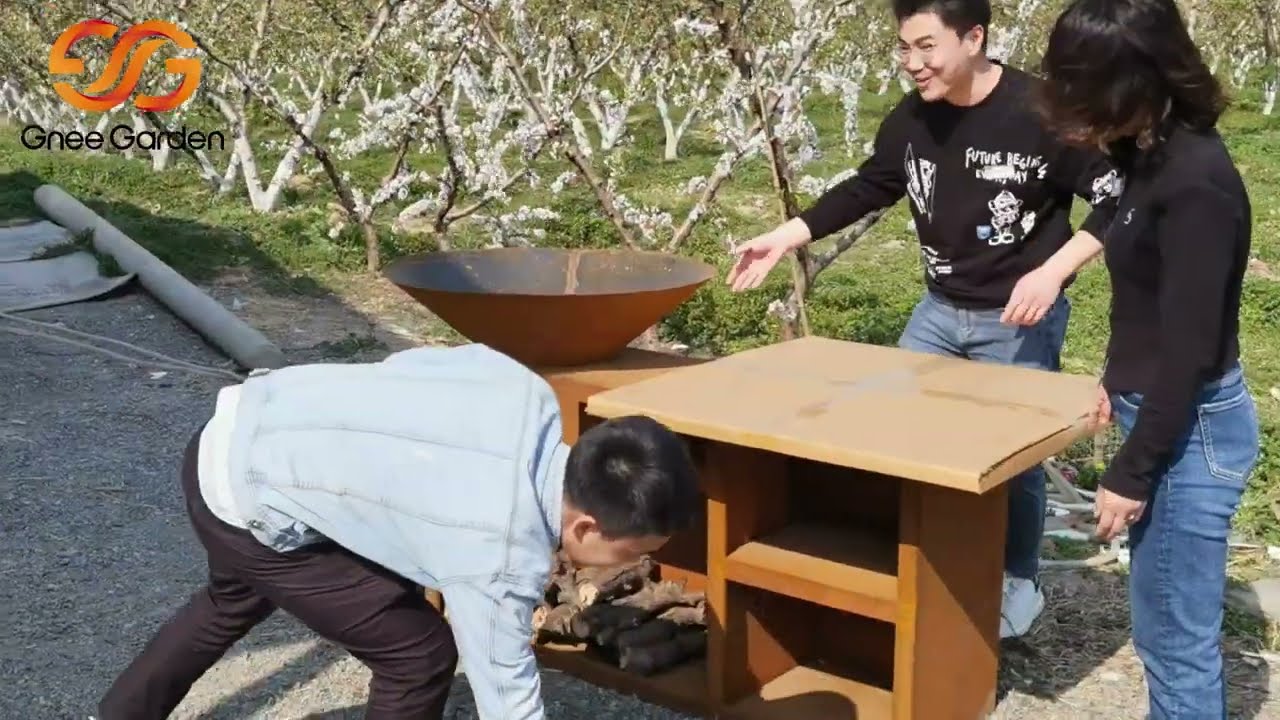In this landscape-oriented color photograph, three individuals, likely of East Asian descent, are setting up an outdoor scene in what appears to be a garden or vineyard. The focal point is a wooden table with a square cardboard box on top, a large red wok on the left, and firewood stacked in a cabinet underneath. To the left of the table is a circular pot. Near this table are trees with white buds, and the background features a green grassy landscape with additional tree-lined fields.

In the foreground, a man in a jean jacket and black pants is kneeling, seemingly about to pick up an item. To his right, a slender woman with dark hair, partially obscuring her face, is wearing a black long-sleeved shirt and blue jeans. Behind them is another man, also with dark hair, wearing glasses, a black long-sleeved shirt, and blue jeans, who is smiling and pointing toward the wok. The top left corner of the image features a logo that reads "GNEE Garden" with two interlocking G's. Their activities suggest they are preparing or assembling something, adding an air of anticipation and communal effort to the scene.